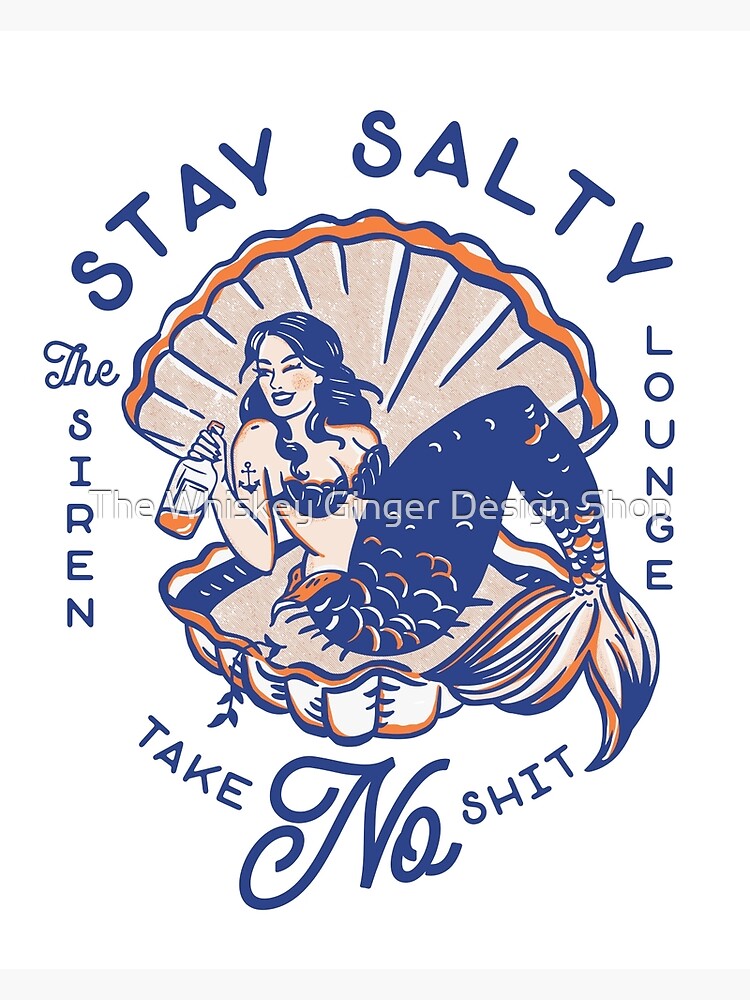This image is a computer graphic design representing a sign and logo for a bar called "The Siren Lounge." The background is white, featuring a watermark that reads "The Whiskey Ginger Design Shop." Dominating the design is an illustration of a smiling mermaid with a large tail, sitting inside a giant beige clamshell with blue and orange outlines. The mermaid is holding a partially empty whiskey bottle and has a tattoo of a sailboat anchor on her bicep. At the top of the image, in blue letters, it says "Stay salty." On the left side of the mermaid, the text reads "The Siren," and on the right, it says "Lounge." Below the clamshell, in blue letters, the phrase "Take no shit" is prominently displayed.